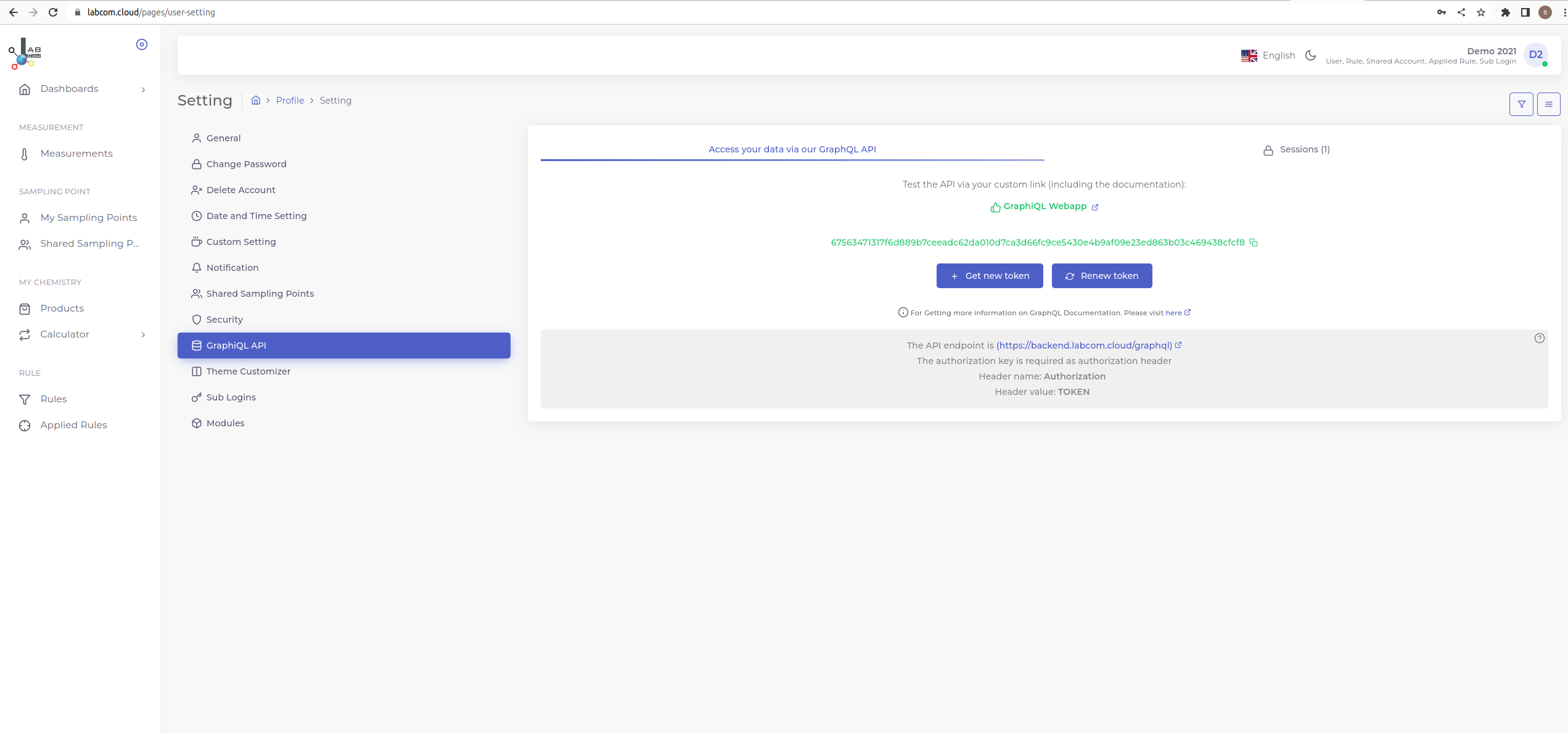The image depicts a desktop computer screen with a predominantly white background. On the left-hand side, a white toolbar is fully expanded, taking up a significant portion of the screen. To the right, a light gray panel serves as the main display area. Above this section, the browser's address bar indicates the user is on the "User Settings" page of labcom.clouds.com, specifically at the URL "labcom.clouds.com/pages/user-settings." 

The settings interface is visible, showcasing options like "General," "Change Password," "Delete Account," among others. Notably, the "GraphQL API" option is highlighted with a prominent blue rectangle, indicating it is currently selected. Adjacent to this, a pop-up window titled "Access Your Data via GraphQL API" presents options for managing access tokens, featuring two blue buttons labeled "Get New Token" and "Renew Token."

The overall context suggests that the user is navigating a settings panel related to an application, focusing on configuring or obtaining access tokens for a GraphQL API.